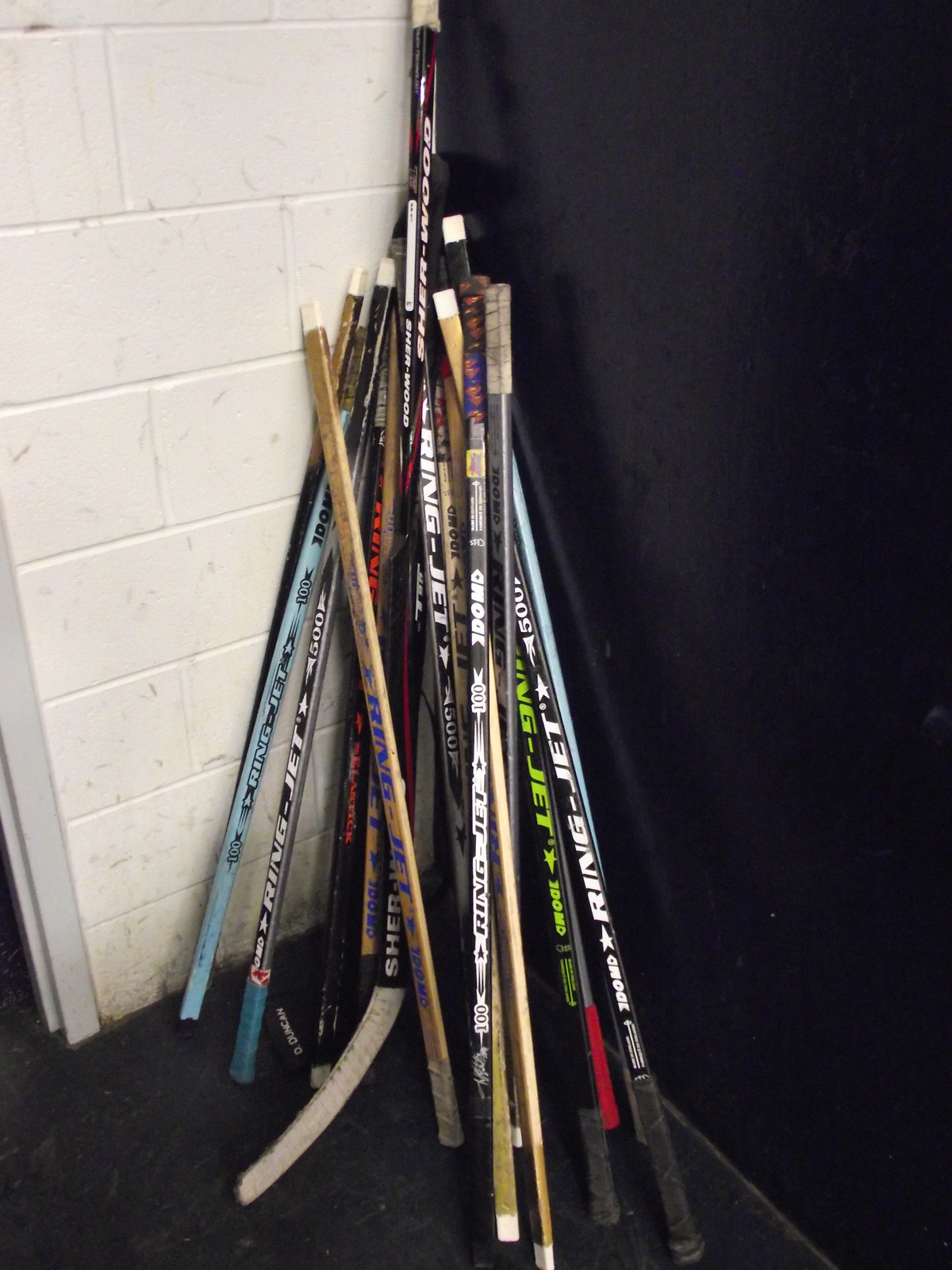The image depicts a corner of a room where two walls meet. One wall is stark black, while the other is made of white rectangular tiled cement blocks with visible scuff marks. Leaning against this corner is a varied collection of approximately 15 to 20 hockey sticks. These sticks come in multiple colors, including blue, black, green, red, white, and brown, and feature different designs and writings, such as "ring-jet" and numbers like "500" and "100." Some of the sticks have the characteristic curved ends commonly found on hockey sticks, while others appear to be straight rods. The floor is black, and on the left side of the white wall, the edge of a door frame is visible, suggesting the presence of a doorway leading to a hallway.